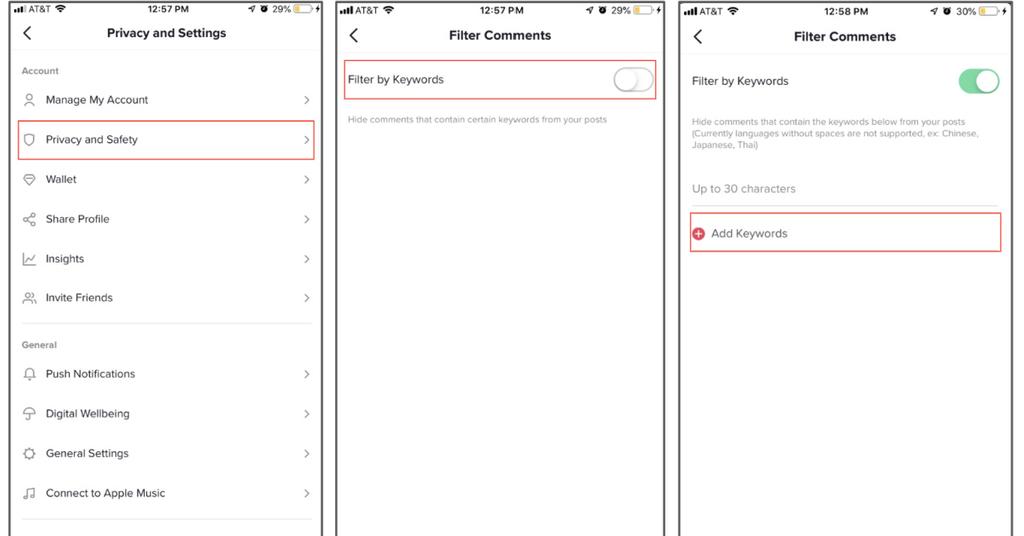The image comprises three distinct panels, each framed with a black trim and possessing either a square or rectangular shape, but lacking a bottom edge. 

**Panel 1 (Left):**  
- The top bar displays the cell signal (AT&T), Wi-Fi signal, and the time (12:57 p.m.), with the battery level at 29% on the right.
- Below, it reads "Status" followed by "Privacy," and "Settings."
- Several sections are listed with right-facing arrows, starting with "Manage My Account," followed by "Privacy and Safety" outlined in red.
- Additional sections include "Wallet," "Share Profile," "Insights," "Invite Friends," and a dividing line precedes "General," "Push Notifications," "Digital Well-being," "General Settings," and "Connect to Apple Music."

**Panel 2 (Center):**  
- The top bar replicates the same information (cell signal, Wi-Fi, time at 12:57 p.m., and battery at 29%), with an addition of a left-facing arrow.
- The central section is designated "Filter Comments," capitalizing both F and C.
- It indicates that "Filter by Keywords" is turned off, highlighted with a red-bordered rectangle.
- Below, there's a description: "Hide comments that contain certain keywords from your posts."

**Panel 3 (Right):**  
- The top bar, identical to the others, shows a slightly different time (12:58 p.m.) and a battery level increased to 30%.
- Like the second panel, the central focus is on "Filter Comments," with the "Filter by Keywords" option turned on.
- The description includes: "Hide comments that contain the keywords below from your posts. Currently, languages without spaces are not supported, e.g., Chinese, Japanese, and Thai, up to 30 characters."
- Below this description, a red banner with a rectangle includes a red circle with a plus sign, accompanied by the text "Add Keywords."

Each panel collectively forms a detailed series of settings and configurations, specifically around account management, privacy, and comment moderation.